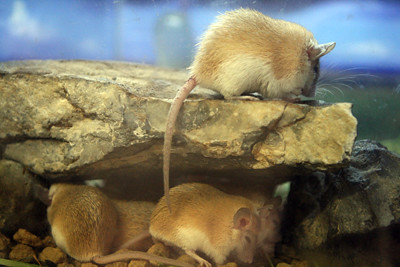This photograph captures a close-up scene of three light to medium beige mice with long, stringy tails, set in a naturalistic enclosure that simulates an outdoor environment. The main focus is a rock structure, likely made of limestone or granite, situated prominently in the center. One mouse is perched on top of the rock ledge, facing away from the camera, with its tail draping over the edge. Below the overhang, two more mice are partially visible—one curled up as if napping, and the other with its back turned. The background features a soft, blurred blue sky with hints of clouds and distant greenery, enhancing the perception of an open and well-kept space. The entire setting looks clean and meticulously arranged to provide a comfortable habitat for these small rodents.